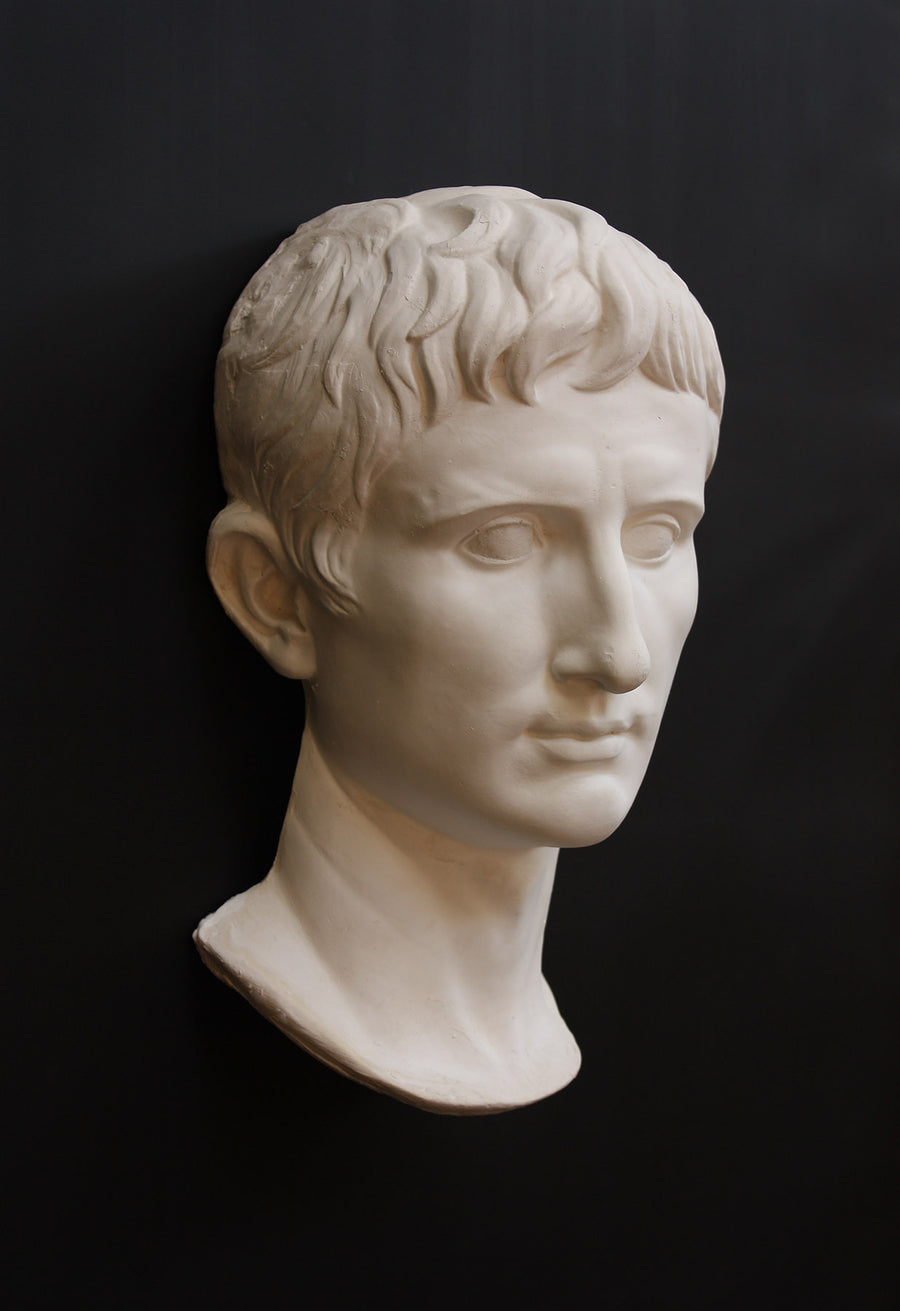The image depicts a detailed bust carving of a historical figure's head and neck, crafted from an off-white, ceramic-like material that resembles white marble or alabaster. The bust features a man with short, coily hair and a well-defined nose, although the eyes are not intricately detailed and appear blank. There is no text in the image, and the backdrop is a solid black, likely a cloth, which creates a stark contrast with the light color of the sculpture. The photograph is presented in a vertically oriented rectangle, focusing closely on the bust without any additional setting or style elements.